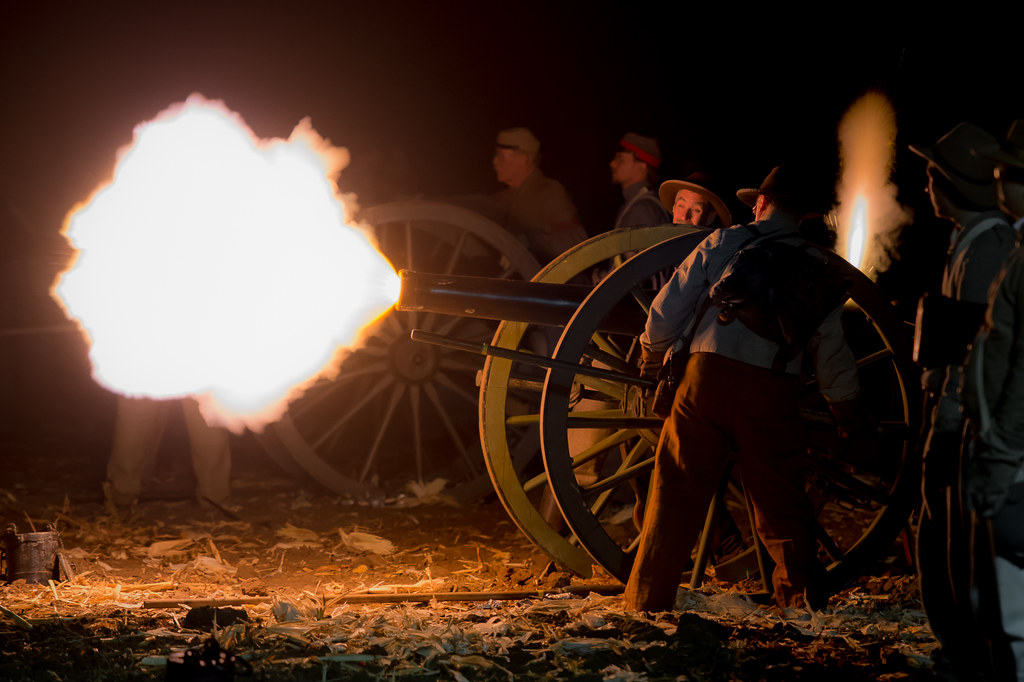This is a full-color, horizontally rectangular photograph taken outdoors at night using natural light, likely by a professional photographer. The scene captures an intense moment of a war reenactment, specifically depicting a Civil War-era cannon firing. The atmosphere is dark, suggesting an open field, with lots of dirt visible around the scene.

At the forefront, an old-style cannon with a large wooden wagon wheel is the main focus. It has just been fired, evidenced by a dramatic burst of fire erupting from its barrel. Flames are also visible from where the fuse was lit, enhancing the realism of the reenactment. Two men, dressed in period-accurate Civil War attire, are stationed on either side of the cannon's wheels, seemingly holding the spokes to control the recoil.

In the background, additional participants in authentic old-time clothing are gathered around other cannons, either participating in or observing the action. Another cannon in the backdrop also shows signs of recent activity with visible flames. The image vividly captures the historical authenticity and dynamic energy of the reenactment.